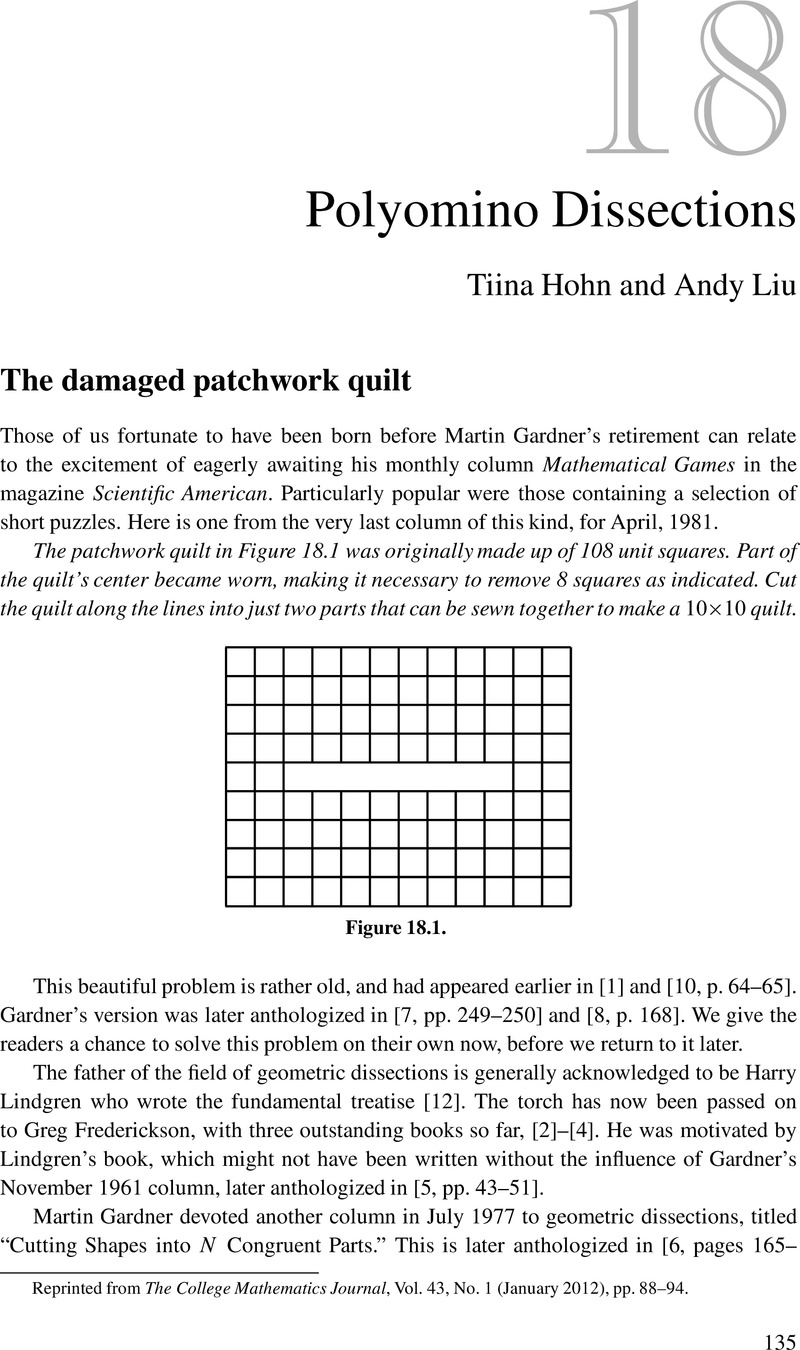The image is a close-up digital scan of a page, primarily consisting of text on a white background in black and light gray font. At the top right of the page, there is a large light gray number "18." Below it, in black font, it reads "Polyomino Dissections" and lists the authors "Tina Hohn" (spelled as Tina with two I's) and "Andy Liu." Following this, there is a bold subtitle "The Damaged Patchwork Quilt." A paragraph beneath the subtitle begins with "Those of us fortunate to have been born before Martin Gardner's retirement can relate to the excitement of eagerly awaiting his monthly column, Mathematical Games, in the magazine Scientific American. Particularly popular were those containing a selection of short puzzles." Centrally, there’s a diagram featuring a square grid with black lines, labeled as "Figure 18-1." At the bottom of the page, there is a citation: "Reprinted from the College Mathematics Journal, volume 43, number 1, January 2012, pages 88 to 94."